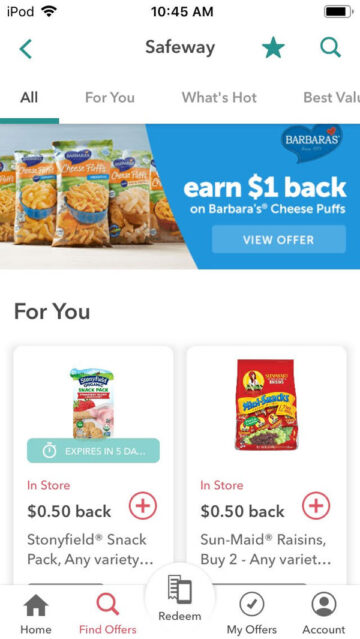The image displays the screen of an iPod, showing an app interface. At the top of the screen, the status bar includes the time (10:45 a.m.), Wi-Fi icon, almost full battery icon, and a notification that the top is at Safeway. There is a star icon, a search button, and a back button also visible.

Below the status bar, tabs labeled "All," "For You," "What's Hot," and "Best Value" are present. Under the "For You" tab, the first offer displayed is for "Barbara's," promising $1 back on Barbara's Cheese Puffs. The offer can be viewed by clicking "View Offer." This deal is characterized by an eye-catching red circle with a plus sign and is set to expire in five days.

Following the Barbara’s offer are additional in-store offers: 
- "Stonyfield Snack Pack: Any variety," promising 50 cents back.
- "Sun-Maid Raisins: Buy two, any variety," also offering 50 cents back.

Each of these offers is accompanied by the same red-circle plus sign to indicate an option to add them to the user’s list. 

At the bottom of the screen, a navigation menu includes "Home," "Find Offers" (highlighted in red, suggesting it is the current section), "Redeem My Offers," and "Account," with the other options displayed in black text.

The user interface features a diverse color palette, incorporating black, green, blue, orange, red, yellow, and brown elements against the background.